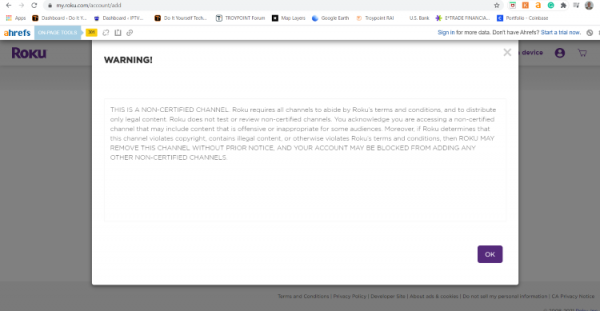The image depicts a complex user interface with a multitude of icons and elements. On the top left, there are arrows pointing left and right, followed by a circular arrow icon within a gray box that features a lock symbol. Adjacent to this, there is an arrangement of various icons: a star, a blue square with an indeterminate middle element, an orange icon, the Amazon logo, possibly within a teal circle, a puzzle piece, and an icon consisting of three lines with a '+' sign. Furthermore, there is a circular icon showcasing a person's face.

In the next row, a series of tabs are visible, with the first one labeled "Apps." There are a total of eleven tabs, although only the first is legible; the remaining ten are indistinct. 

Underneath these tabs, there's a prominent banner that appears to read "AHREFS," where the letter 'A' is in orange, and the other letters are in blue. To the side of this, there's a blue tab accompanied by something that resembles a yellow box, though the icons are not clearly identifiable. To the far right, there might be a login section.

Additionally, a pop-up appears on the interface, serving as a warning. This warning message comprises six lines of text. In the bottom right-hand corner of the pop-up, there's an "OK" button within a purple rectangle featuring white text.